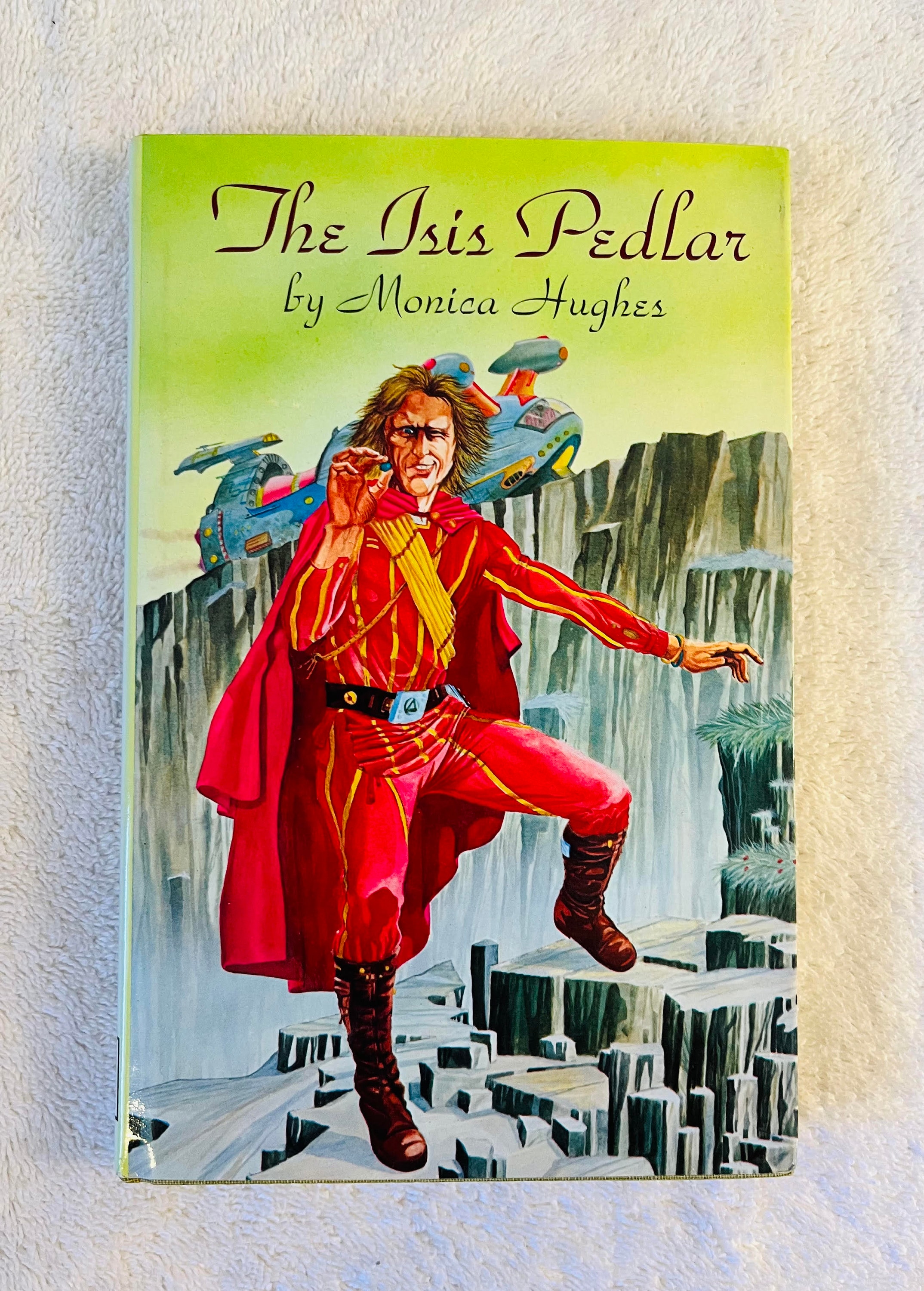This is an image of a children's hardcover book titled "The Isis Pedlar" by Monica Hughes. The book is predominantly green, with a lime green hue. The cover illustration is vibrant and detailed, featuring a man in a bright red, full-body outfit with yellow highlights. He sports a red cape, a black belt with a white buckle, and tall black boots. The man has long brown hair, is grinning, and squinting one eye as he climbs up a mountainside. Behind him, a blue spaceship is visible against the rocky mountain background, hinting at an adventurous storyline.